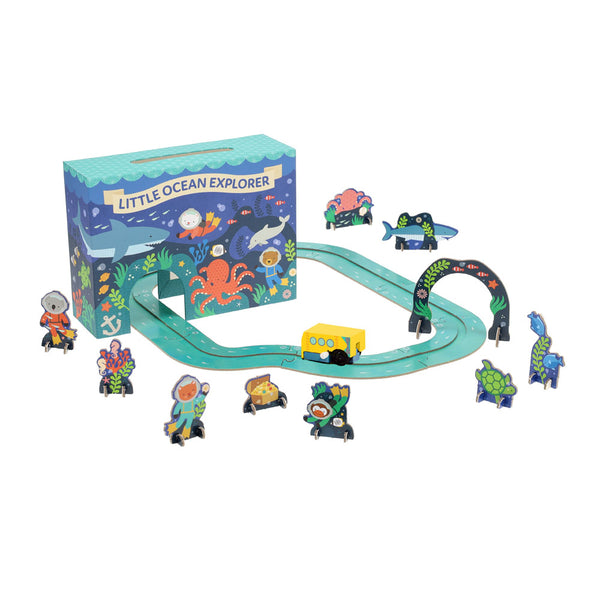The image depicts a vibrant, full-color playset titled "Little Ocean Explorer." The playset features a blue cardboard track designed for a small yellow vehicle to navigate. The track goes under a colorfully illustrated archway and a box adorned with lively ocean-themed graphics, including sharks, a red octopus, various fish, and aquatic plants. Surrounding the track are ten standing cardboard characters, which include a scuba-diving child and bear, a koala in scuba gear, a diver, a treasure chest, fish, a turtle, a blue shark, coral, seahorses, and potentially a pink squid. This playful scene captures an engaging underwater adventure, showcasing the interactive and imaginative elements of the toy set.